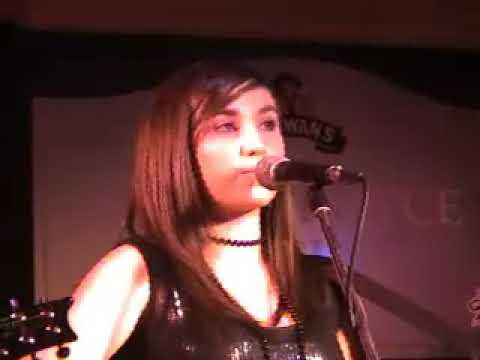The photograph captures a woman with lighter skin and straight brown hair, singing on a dimly lit platform or stage. Her hair is styled with bangs pulled to the side and tucked behind her ear, while the rest cascades onto her shoulders. She is wearing a black tank top and an elegant black beaded necklace that wraps around her neck twice, with one row sitting high and the other draping across her bust. In front of her is a microphone, and she appears to be looking out towards the audience with her mouth closed. The background features a white board with a partially visible logo ending in "W-A-N-S" and a black border. There is a purplish-red haze due to the lighting. On the lower left corner of the image, the headstock of a guitar is partially visible. The photograph is of poor quality with a slightly blurry and dim appearance, suggesting it might have been taken indoors under less-than-ideal lighting conditions.